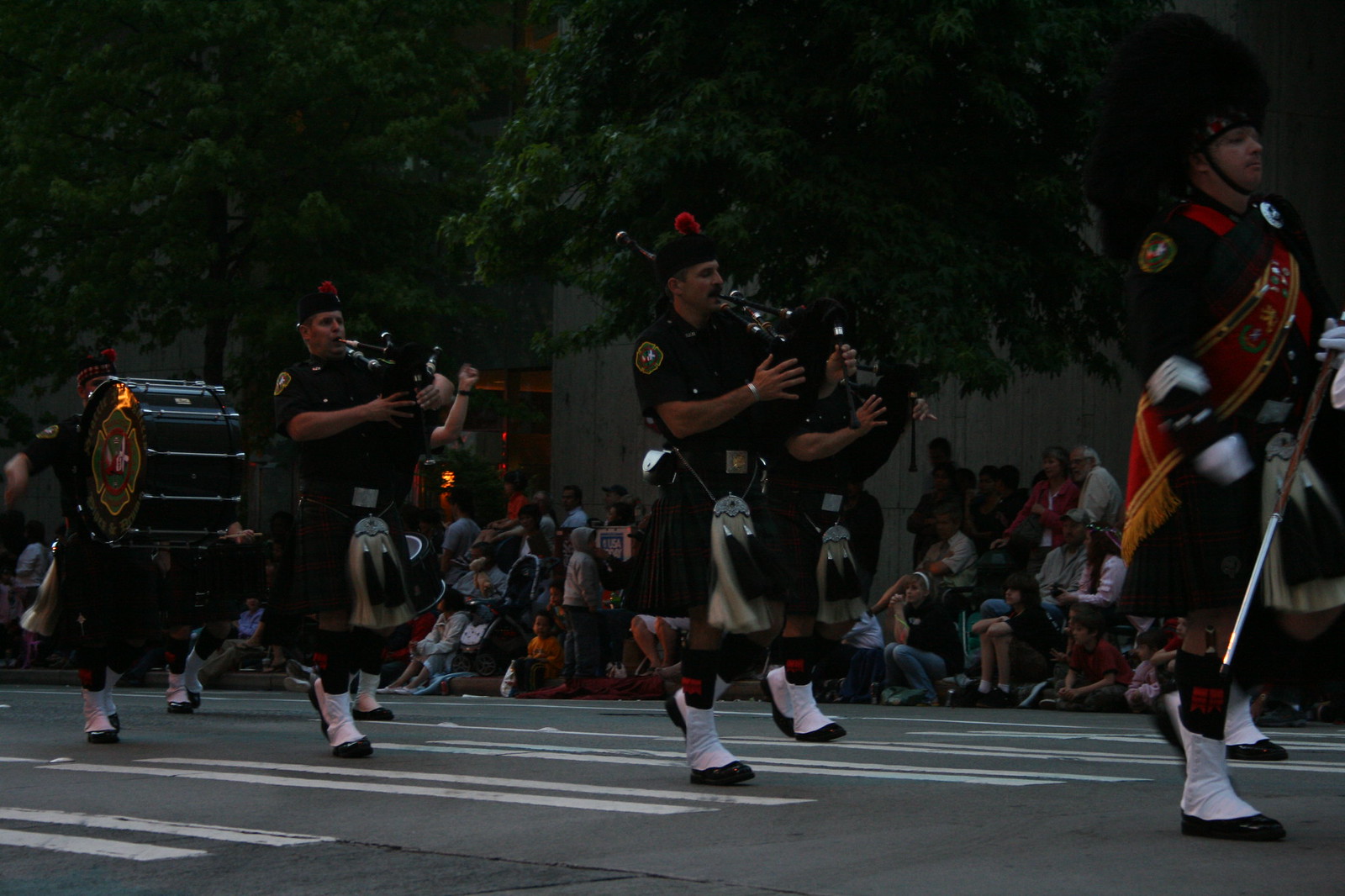This is a dark, color photograph in landscape orientation, depicting a lively parade scene. The image features three bagpipers and one drummer marching towards the right on a street marked with a zebra crossing. The Scottish musicians are adorned in traditional kilts, white socks, and black and white shoes, along with black caps featuring red feathers. A noteworthy detail is the drummer positioned on the left, who is carrying a large drum. The scene is set either at night or near dusk, adding to the overall dimness of the image. In the background, a crowd of onlookers can be seen lining the street; they are either standing, sitting on the curb, or positioned on chairs, attentively watching the parade. Just barely visible in the darkness are some trees, contributing a touch of natural foliage to the scene. The photograph captures a moment of photographic representational realism, focusing on the traditional Scottish elements and the parade atmosphere.